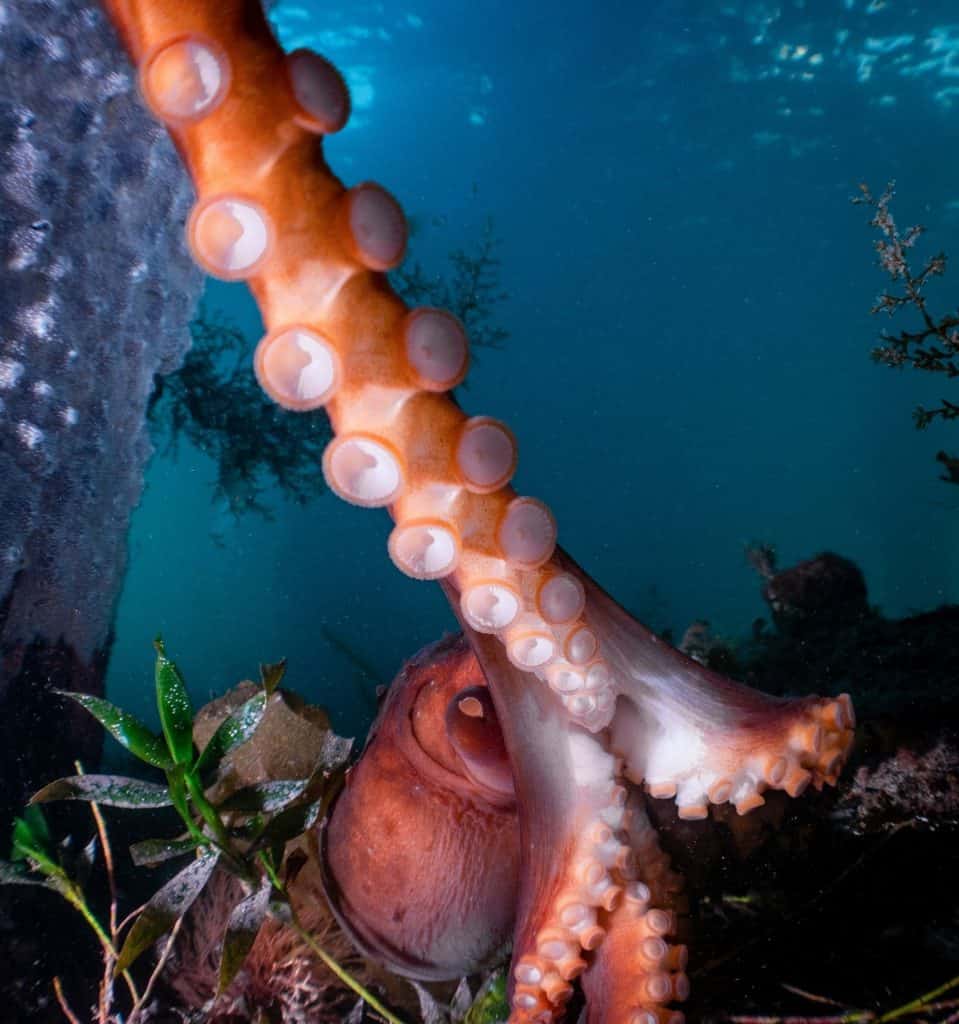The photograph captures a vivid underwater scene, focusing primarily on a bright orange and white octopus. At the center of the image, a large tentacle stretches diagonally from the bottom right to the upper left, bringing its circular white suction cups into sharp focus close to the camera. The octopus's head, along with a couple of other tentacles, is visible behind the prominently featured limb, displaying a beautiful blend of orange and reddish hues. The backdrop reveals an underwater setting about 30 to 40 feet below the surface, illuminated by a gradient of medium to lighter blue tones indicating the water's depth and surface reflection. Surrounding the octopus, various aquatic life forms can be seen, including green stem plants with leaves and a coral patch located in the lower left. Additionally, a gray stone wall or rock structure provides contrast on the left side, enhancing the diversity of the underwater landscape. The lower right side fades into a shadowy area, adding depth to the scene.